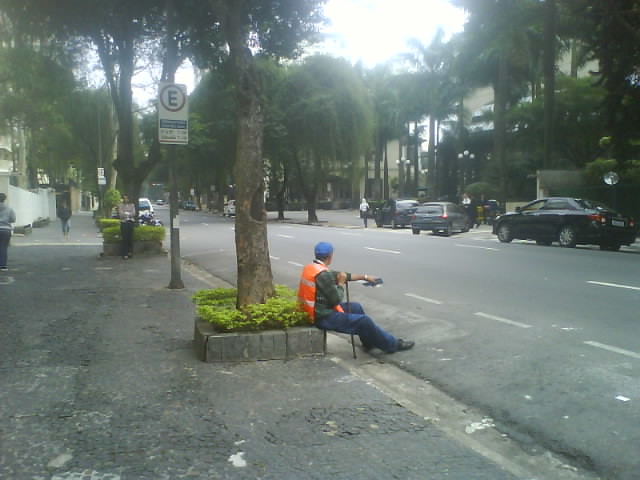The image depicts a tranquil street scene centered around a man sitting on a tree planter along a wide, tree-lined sidewalk. The man, dressed in an orange construction vest over a green shirt and blue jeans, sports a blue hat and appears to be holding a cane in his right hand, with a gold wristwatch on his left wrist. His left hand is extended, potentially holding a piece of paper. The planter he sits on is surrounded by light green plants and bordered by squarish concrete blocks. Behind him, the road remains mostly empty with some parked cars visible, predominantly black or gray hatchbacks. Along the sidewalk, there are multiple trees with bases wrapped in shrubbery, including coconut and other tropical trees. A street sign marked with an 'E' enclosed in a circle is situated to his left. Across the street, more cars are parked and a few people can be seen walking or tending to their vehicles. The street itself is dark gray, featuring three lanes, and the entire scene is bathed in daytime sunlight, giving it a peaceful, sunlit ambiance.